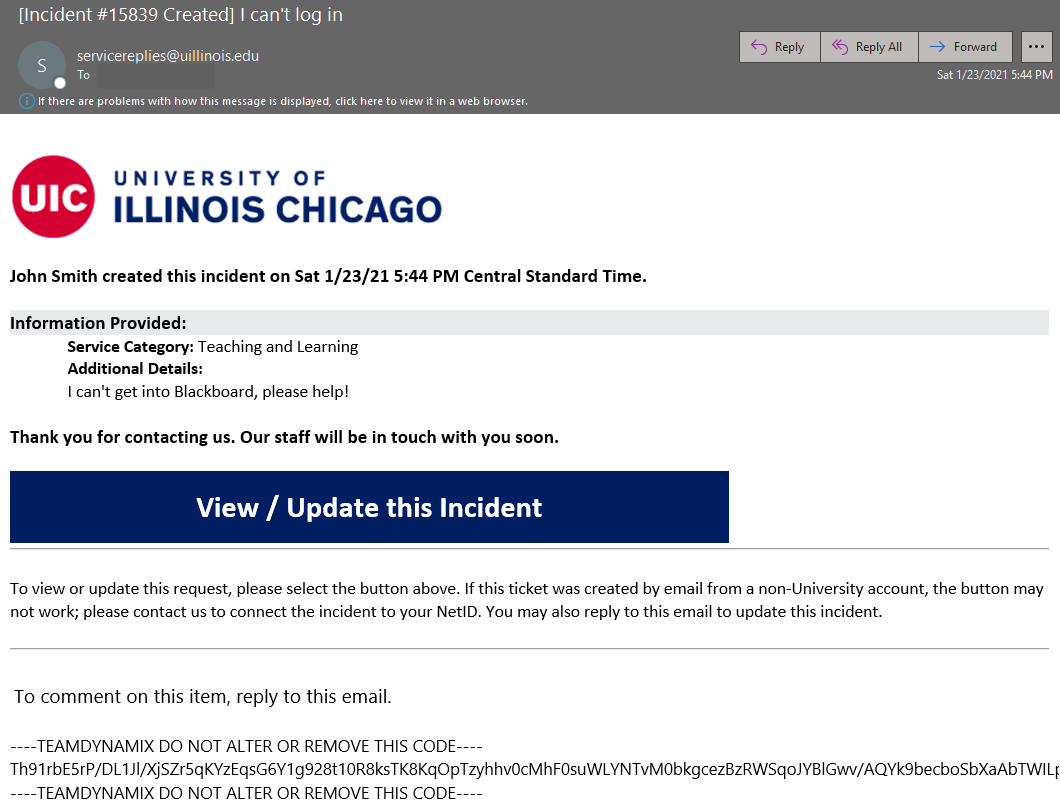The image features an email notification from the University of Illinois Chicago in response to an incident report. 

At the top, "University of Illinois Chicago" is prominently displayed in dark blue, with "Illinois Chicago" slightly larger and also in blue. Below this, a red round circle houses the acronym "UIC" in white. Above the circle, there's a dark gray banner that reads "Incident Number 15839 Created," with the issue "I Can’t Log In" noted next to it. 

The email is from "service replies" at "uillinois.edu," and nearby, a small gray circle contains a white "S" with a tiny white dot beneath it. An informational message advises, "If there are problems with how this message is displayed, click here to view it in the web browser."

On the right side, options to "Reply," "Reply All," and "Forward" are shown on gray banners with arrows: a purple arrow pointing left for the first two and a blue arrow pointing right for "Forward." 

A timestamp below these options states, "Saturday, 1/23/2021, 5:44 PM." The individual's name, "John Smith," indicates that he created this incident at the specified time (Central Standard Time). The incident details mention, "Service Category: Teaching and Learning," with the issue outlined as, "I can't get into Blackboard, please help."

A closing note offers thanks, stating, "Thank you for contacting us. Our staff will be in touch with you soon." A navy blue banner below invites users to "View/Update This Incident." 

Further instructions on a white background explain, "To view or update this request, please select the button above. If this ticket was created by email from a non-university account, the button may not work. Please contact us to connect the incident to your Net ID. You may also reply to this email to update this incident." 

A fine gray line separates these details from additional text, which reads, "To comment on this item, reply to this email." The message concludes with a caution not to alter or remove coded information by "TeamDynamix," followed by a series of black text codes.